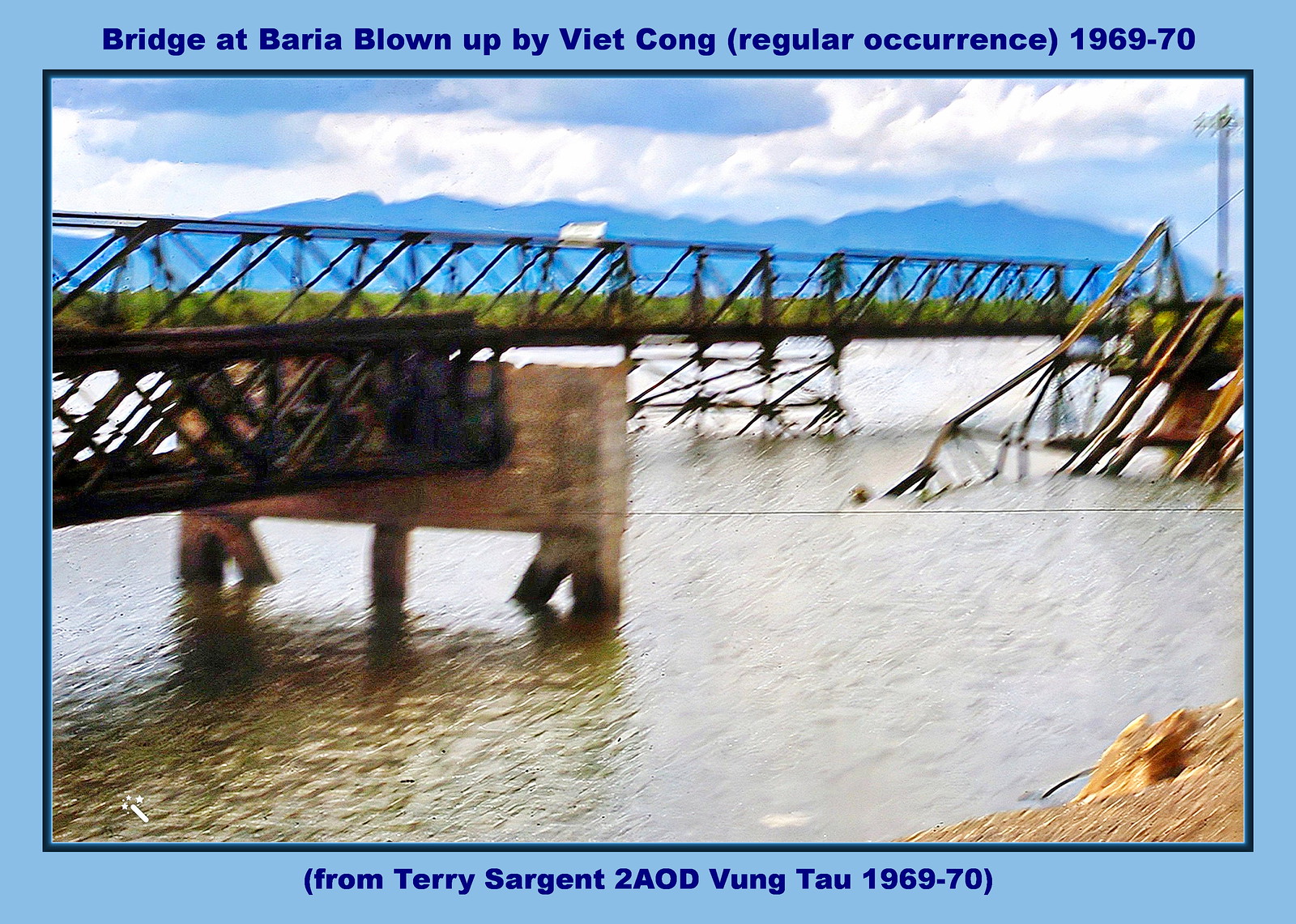In the image, a color photograph taken during daylight and framed by a blue border, depicts a scene of two metal bridges over a large, muddy brown river. The photograph is accompanied by dark blue text along the top border, stating: "Bridge up area blown up by Viet Cong, regular occurrence 1969 to 70." At the bottom, it reads: "From Terry Sargent to AOD Vung Tau, 1969 to 70."

The picture, somewhat blurry and seemingly taken from a moving or out-of-focus camera, shows the bridges running parallel to each other from a side and back angle. The nearer bridge has a section that abruptly cuts off on the left, indicating that it has been destroyed, with remnants dropped into the river. The concrete section in the middle stands amid the destruction. The second bridge in the background remains intact.

The surrounding landscape features a muddy, rocky riverbank with a tall blue mountain range and patches of greenery under a partly cloudy sky, adding depth to the depiction of the scene.